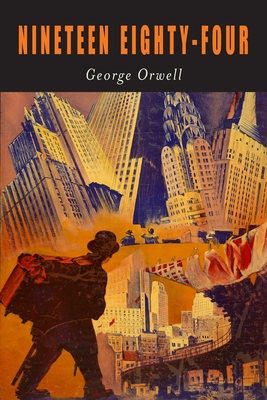This is the cover page of George Orwell's book, 1984, depicted in a painted and somewhat futuristic style. The top portion features a black horizontal strip, with "1984" prominently written in large orange text and the author's name, "George Orwell," in smaller white text, both set in different fonts. Below this strip, the cover showcases a surreal and slightly chaotic drawing of a cityscape with cream-colored buildings, skyscrapers, over bridges, and soldiers, giving it a dystopian feel. The city's silhouettes appear slanted and disorganized, almost collage-like. In the bottom left corner, there is a silhouette of a man wearing a hat, seemingly in uniform and possibly carrying a gun, walking towards the city with a big red bag on his back. The overall color scheme is dominated by dark tones, with prominent yellow and orange hues accentuating the scene, adding to the dystopian atmosphere.